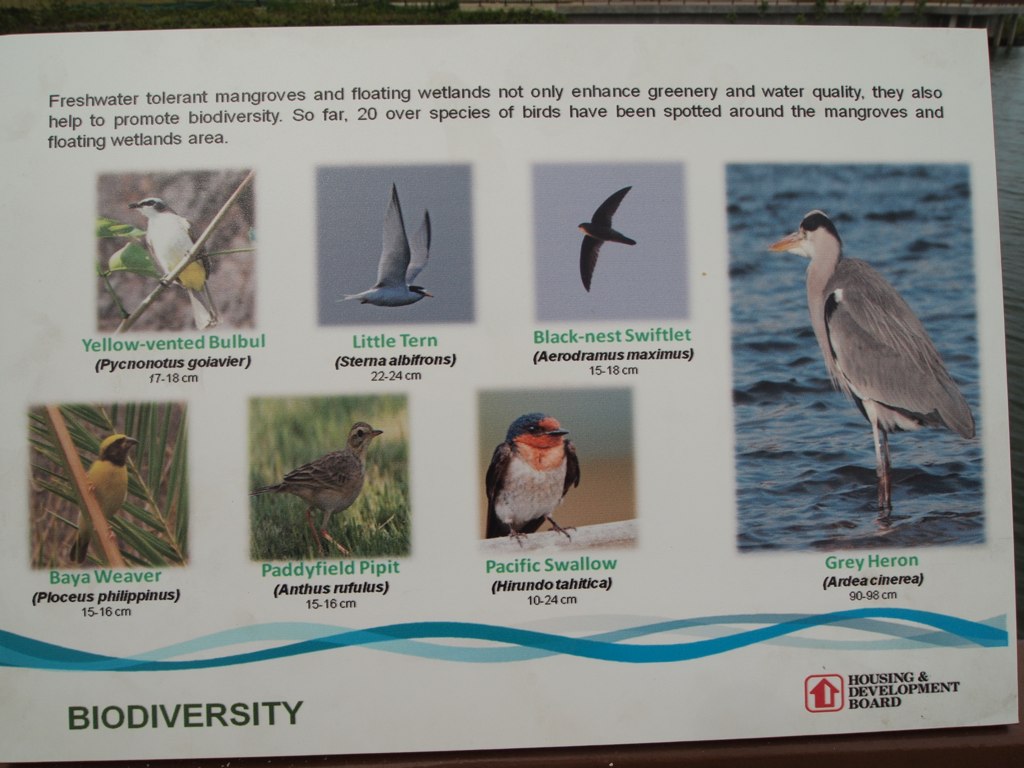This detailed informational sign, likely found outdoors, promotes the biodiversity benefits of freshwater-tolerant mangroves and floating wetlands. The white background features prominently at the top an informative paragraph explaining that these natural features not only enhance greenery and water quality but also support biodiversity, noting that over 20 species of birds have been observed in the area.

Centrally displayed are seven bird photographs: six smaller square images, each with a different bird and annotated with the bird's name and measurements. The birds include the yellow-vented bulbul, little tern, black-nest swiftlet, baya weaver, paddyfield pipit, and Pacific swallow. To the right of these smaller images is a larger photograph of a grey heron standing upright in water, with dimensions noted as 90 to 98 centimeters.

At the bottom of the sign, in bold black lettering on the left, the word "Biodiversity" is displayed. The bottom right corner features the logo of the Housing and Development Board, represented by a red upward-pointing arrow. A blue ribbon stretches along the bottom edge, adding an aesthetic touch to the informative display.